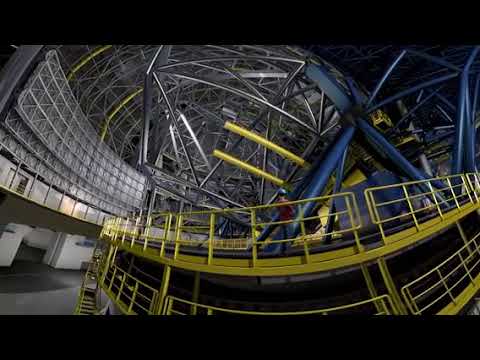The image depicts the interior of an industrial facility with a fishbowl-style camera effect creating a rounded perspective. The ceiling is a complex web of thin silver and metal scaffolding and support beams. The walls are lined with flat white beams and additional scaffolding. The lower part of the walls, which are painted white, features a small opening leading into another hallway. The center of the image is dominated by multi-floored scaffolding with yellow railings and black flooring. Large blue support pillars extend from the top of the scaffolding. In the midsection of the scaffolding, a person stands, wearing blue jeans, a red long-sleeve t-shirt, and a blue hard hat. They appear to be looking down towards the camera. The floor, visible in the lower left-hand corner, is bare gray concrete. The intricate, multi-colored metalwork gives an impression of organized yet chaotic entanglements, typical of a factory or metalworking facility.